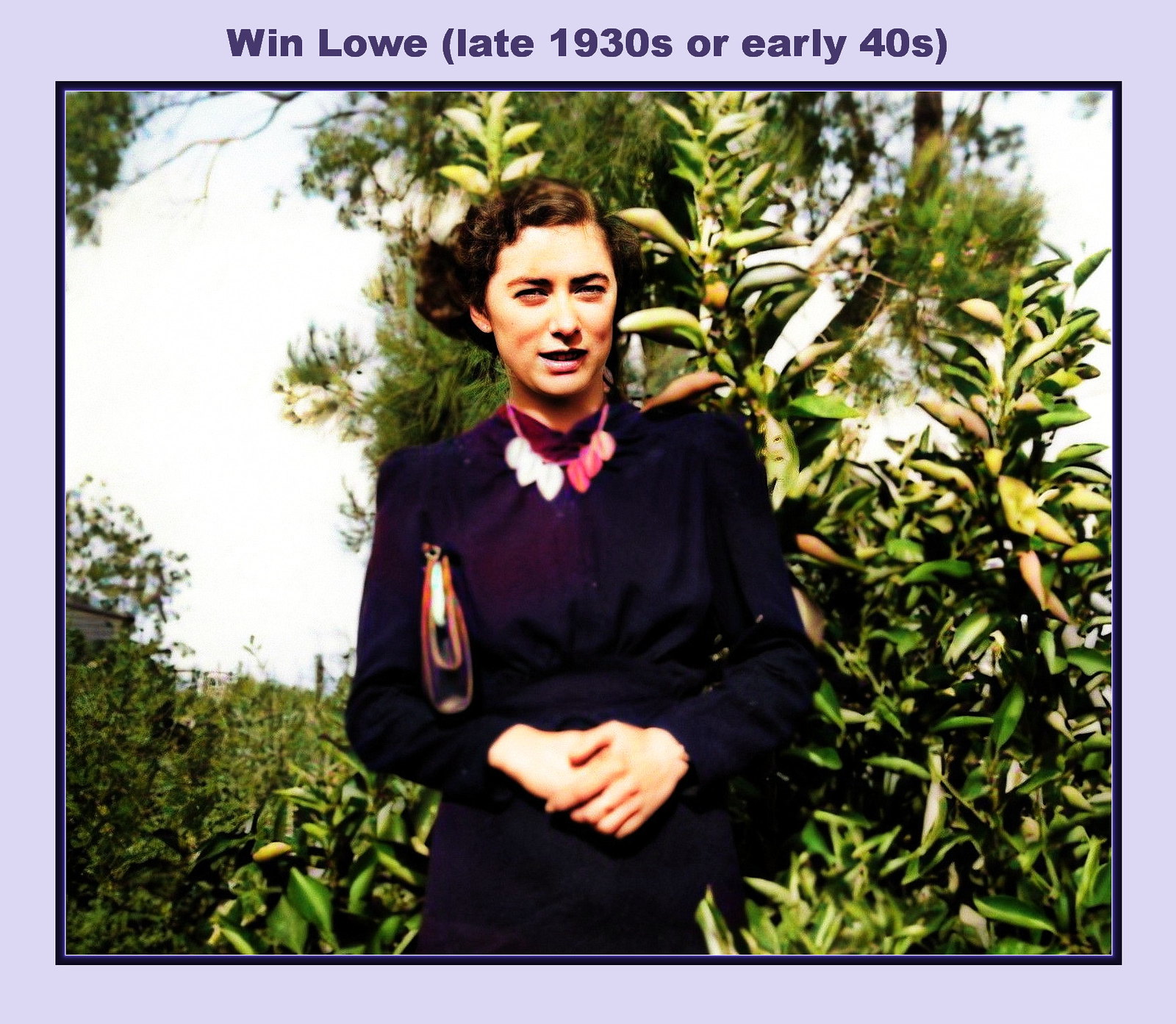The photograph, almost square in shape, is bordered by a light bluish-purple frame with a narrow black inner border. At the very top, in purple text, it reads, “Minn Low, late 1930s or early 40s.” In the center of this composition is an image of a woman posed from the hips up. She is dressed in a long-sleeved dark blue or navy dress that covers her wrists and neck. Around her neck, she wears a necklace adorned with white and pink charms or beads. Cradled under her right arm is a brown clutch purse, while her hands are clasped together, resting at her stomach. The woman's short, curly brown hair frames her face, and she is smiling softly, though her eyes are mostly closed. The background showcases a natural setting dense with foliage, leaves, and trees, with a patch of light blue, whitish sky peeking through. This detailed setting suggests she is outdoors, enveloped by nature.